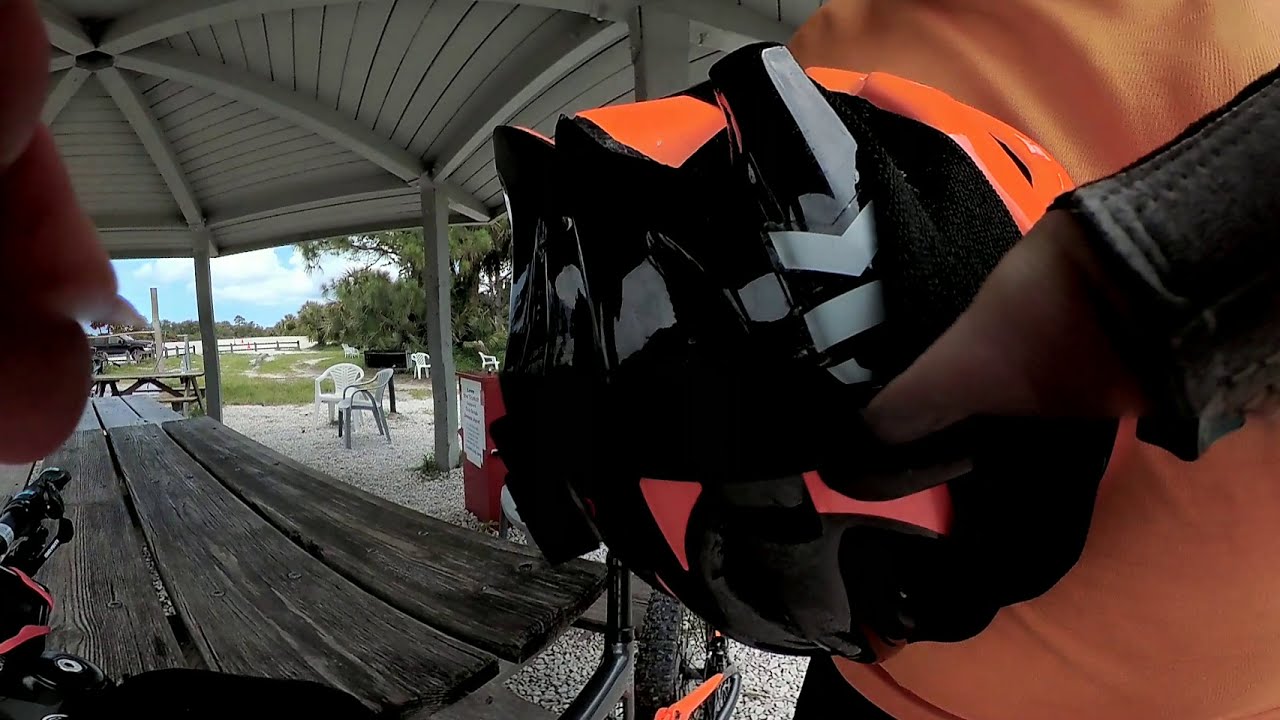In the image, a technologically advanced helmet dominates the center, gripped by someone wearing black gloves and a black leather jacket. The helmet, featuring an orange crest and forward-facing cameras, suggests it's used in a competition. This individual stands under a gazebo-like structure made of gray wooden planks. In the bottom left corner, a wooden picnic table sits on a light gray stone-pebble floor beneath the shading canopy. The background reveals light-colored patio chairs scattered across a green lawn, framed by trees, and under a light blue sky with white clouds. The image is characterized by colors like brown, gray, orange, black, silver, and light blue.